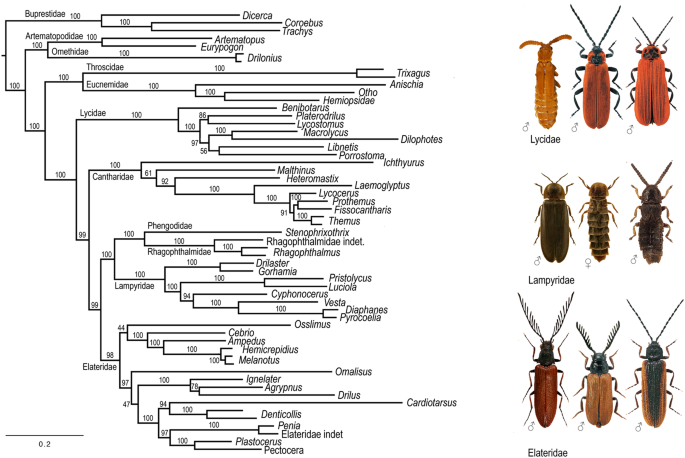The image appears to be an intricate, detailed illustration likely sourced from a scientific textbook, featuring a comprehensive chart on the left and rows of various beetles or insects on the right. The left side of the image showcases a complex diagram depicting the evolutionary relationships and classifications among different insect taxa, resembling a genealogy chart with black branching lines that bifurcate multiple times. Each branch and node is meticulously labeled and numbered, although the text is minuscule and illegible.

Positioned on the right side of the image are three rows of insect illustrations, each row containing three different specimens. The top row displays three orangey rust-brown insects, each with prominent antennae and likely labeled with their specific classifications, albeit the labels are blurred and unreadable. The middle row presents three brown insects adorned with yellowish highlights around their legs and necks, also equipped with antennae and a set of six legs. The bottom row features an orange insect flanked by two yellow insects, all characterized by black heads and noticeably longer, thicker antennae, completing their six-legged anatomy.

Small, barely legible text in the lower-left corner of the chart possibly provides further explanation of the depicted evolutionary links and classification details.